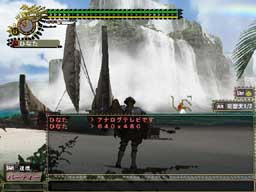In this still from a computer game, a character is standing on a gray surface. Superimposed over the character is a red-colored chat box or player information panel. At the bottom of the screen, there is a gray band, likely containing unreadable information due to its small size. 

The focal point of the background is a massive mountain with multiple cascading waterfalls, with jagged rocks protruding from the flowing water. The sky above is a bright blue scattered with some clouds. On the right side of the image, a palm frond enters the frame, adding to the scenic environment. 

In the top left corner, there is a logo featuring a circle with sun rays, although the details are not clearly visible. Additionally, a yellow and green strip extends two-thirds across the top of the screen, which presumably indicates player health or status.